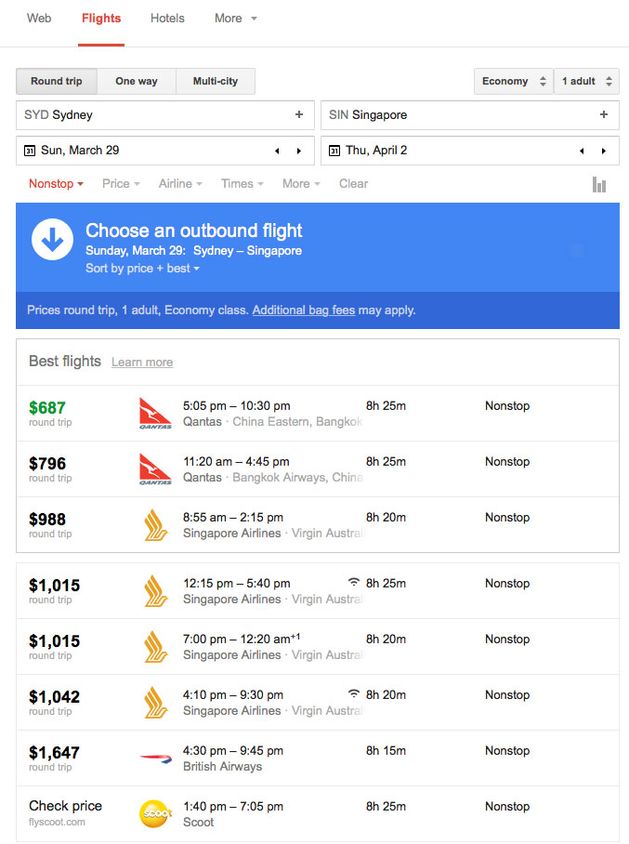The image depicts a tablet screen displaying a flight booking website. The top of the webpage prominently features the heading "Choose an Outbound Flight," while the itinerary shown is from Sydney to Singapore. The travel dates specified are from Sunday, March 29th to Thursday, April 2nd, for a round trip. The very top of the web page includes tabs labeled "Web," "Flights," "Hotels," and "More," but no specific website or app is identified.

Displayed flight options include various airlines, such as Qantas, Singapore Airlines, Scoot, and British Airways, with prices listed from lowest to highest: $687, $796, and $998, respectively. These flights are non-stop, economy class, round trip tickets for one adult. Additional notes mention that extra baggage fees may apply if more luggage is brought.